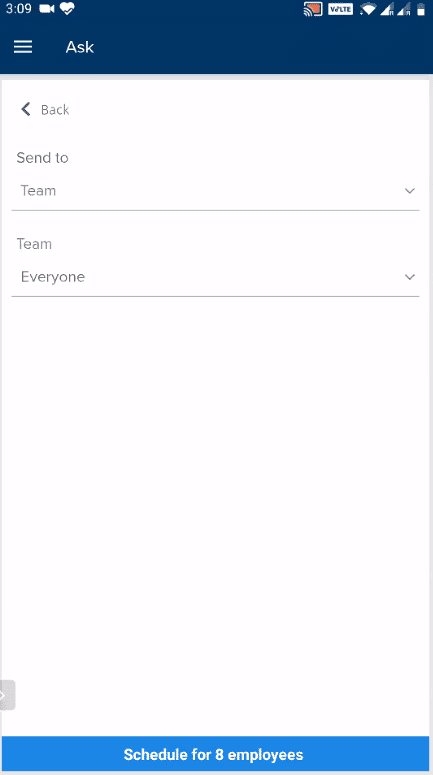The screenshot displays a user's phone screen, specifically while they are navigating a work-related application. The phone status bar at the top right reveals a battery level at approximately 50%, two cellular signal strength indicators—one with a single bar and another with three bars, and a Wi-Fi signal that is nearly full. On the top left, the time displayed is 3:09, alongside icons for video recording and a heart.

In the top center, the word "Ask" is prominently featured in white text against a dark blue background, accompanied by a hamburger menu icon on its left. Directly beneath this area, there is a "Back" button with a leftward-pointing arrow. Below, two categories are visible: "Send to" and a corresponding search field labeled "Team" with a downward arrow.

Further down, another search field marked "Everyone" with a downward arrow appears under the "Team" section. Finally, at the base of the screen, a blue rectangular button displays the text "Schedule for 8 employees" in white.